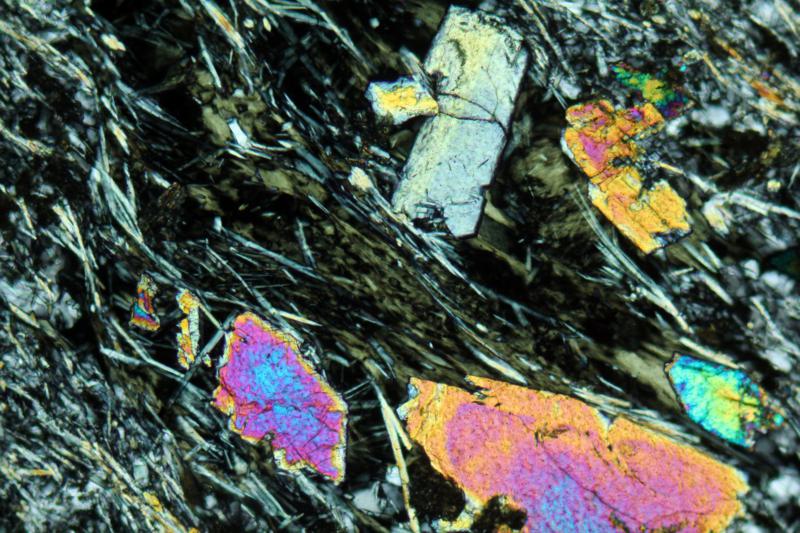A detailed image, reminiscent of a microscopic view, reveals a vibrant and complex scene dominated by an array of abstract, blob-like shapes and intricate strands. The foreground is textured with long, grass-like fibers that weave through the composition, creating a nest-like structure. Scattered throughout are six large, colorful shards, each exuding a unique blend of colors. The central shard transitions from purple to orange and yellow, while others display hues ranging from pink and blue to yellow and green. The background, heavily saturated in greenish-black tones, contrasts sharply with the bright, varied colors of the blobs, which include gray, orange-yellow, and blue shades. Overall, the image evokes a sense of biological or natural complexity, reminiscent of either an illuminated microscopic slide or an infrared photograph of forest foliage interspersed with rainbow-colored elements.